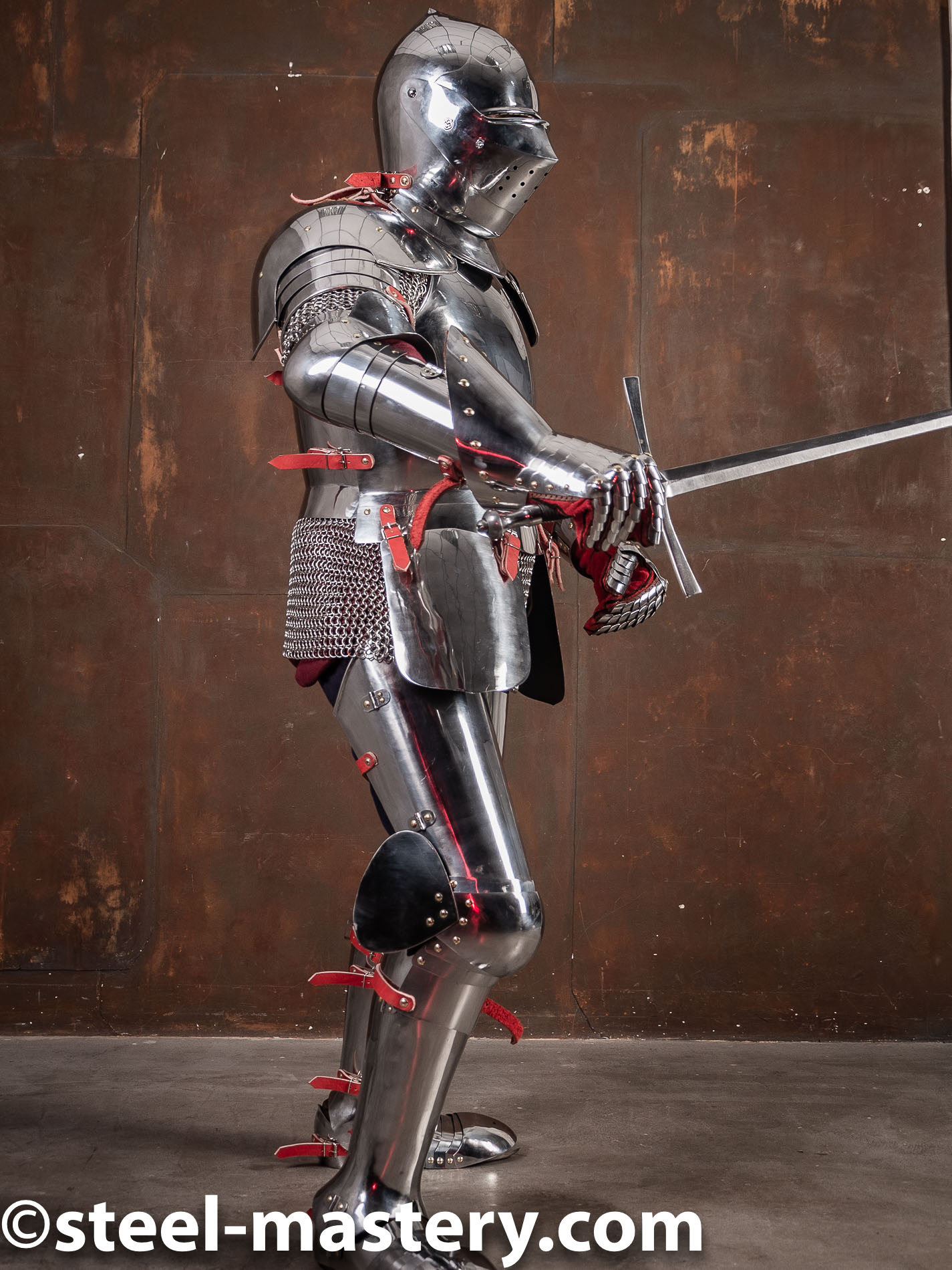This photograph features a medieval knight in gleaming, full body armor, standing on a concrete surface against a plain brown wall. The knight, adorned in intricate metal gear covering from head to toe, holds a metal sword in its right hand. The armor is meticulously detailed, including chainmail visible beneath the metal plates. Red straps are prominently featured, securing various metal components together. The knight's helmet is closed, adding to the authenticity of the historical depiction. An inscription at the bottom reads "steel mystery.com."